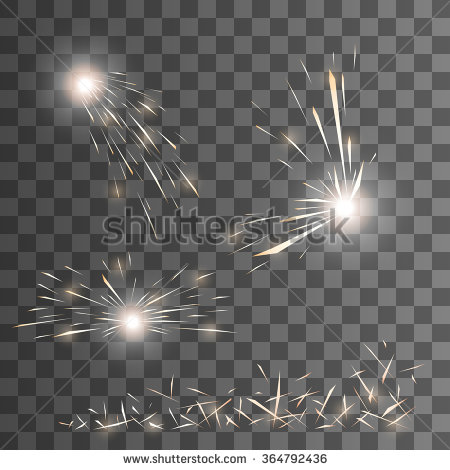The image features a dark gray and light gray checkerboard background that dominates the scene. Amidst this checkerboard pattern, there are three bursts of light resembling sparklers: one situated at the top left, another at the bottom left, and the third at the center right. Additional smaller sparks are visible near the bottom of the image. Centrally overlaid is a Shutterstock watermark, with the text "www.shutterstock.com" and the identifier number "364792436" in small black font at the bottom.